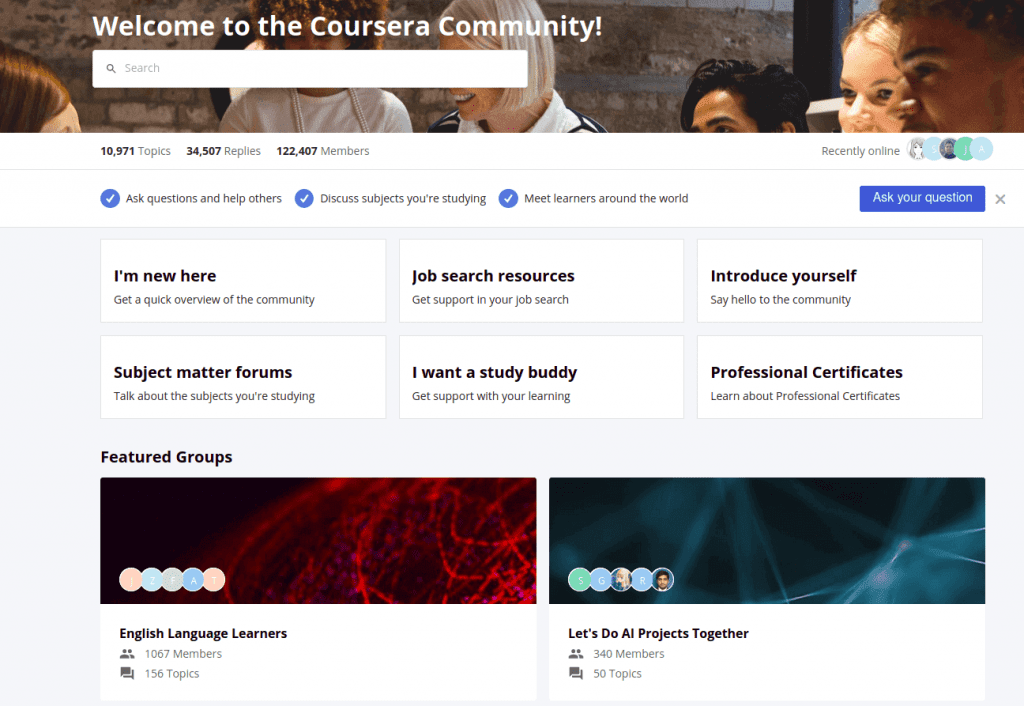This screenshot appears to have been taken from a webpage of a community college or university. On the right-hand side, a group of diverse individuals is featured prominently near the camera. Among them, an African American man with short, curly hair stands beside a Caucasian woman with blonde and brown hair. Nearby, an olive-skinned individual with short, slightly curly hair combed to both sides is partially cut off in the photograph. In front of this person, there is a bleach-blonde woman wearing a white shirt, although her face is obscured by a search bar. She is smiling and laughing, displaying her white teeth. Next to her, an African American woman with curly hair that has gold and brown hues is seen wearing a thin white fleece jacket over a white undershirt.

The wall behind these individuals is a mix of tan and brown colors. On the far left, a light-skinned person with dark brown hair is visible. There's a white rectangle overlaying part of the image, displaying the word "Church" in faded gray with a faded gray magnifying glass icon next to it.

In the webpage's left-hand panel, a series of prompts and check-marked circles are listed:
- "Ask questions to help users."
- "Discuss subjects you are studying."
- "Meet learners around the world."

Below these prompts are six rectangular sections, each with a bold headline followed by regular text:
1. "I'm new here. Get a quick overview of the community."
2. "Subject Matter Forums. Talk about subjects you are studying."
3. "Job Search Resources. Get support for your job search."
4. "I want to study buddy. Get support with your learning."
5. "Introduce yourself. Say hello to the community."
6. "Professional Candidates. Learn about professional certificates."

At the bottom, there are two videos or forums. One of them shows a close-up of red wires and other components, with the caption underneath reading "English Language Learners, 1067 members, 156 topics." On the right-hand side, a title in cyan blue, dark blue, and black reads, "Let's do an iProject together."